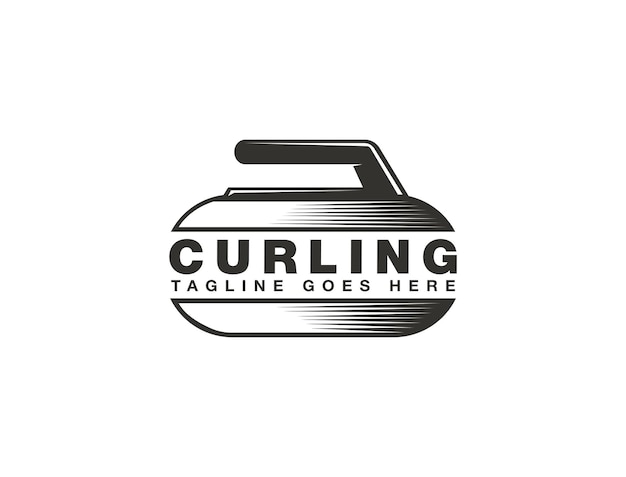This black-and-white logo features a bold, block-style text centered in the middle, reading "Curling," with the placeholder text "Tagline goes here" beneath it. The text is set within an oval-shaped object that resembles a cross between two hamburger buns and a traditional curling iron. On top of this oval sits a distinct black handle, similar to that of an iron or teapot, designed for easy gripping. The oval object itself is adorned with horizontal black and white streaks that gradient from right to left, adding a touch of visual texture to the overall stark design, which stands out against a plain white background.